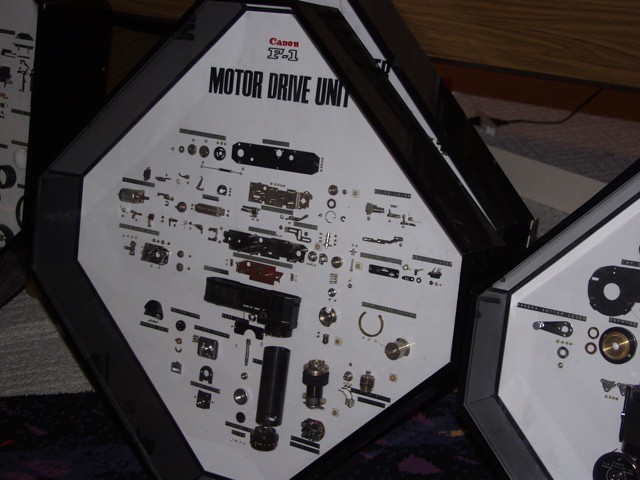This photograph, taken with flash, vividly captures a meticulously arranged display of mechanical components. Dominating the image is a white diamond-shaped mount, edged with a prominent, tall black frame that extends outward significantly. At the top of this mount, bold black letters spell out "Motor Drive Unit," while the iconic red "Canon" logo, accompanied by "F-1", is positioned just below. The white background within the frame is densely adorned with a variety of small metallic pieces, including gold and silver switches, nuts, bolts, and straight metal components. Each piece, varying in size from very tiny to somewhat larger, appears to represent every constituent part of a complex machinery. Behind and to the right of the central display, a similar object can be partially seen, suggesting multiple layers or a depth to the arrangement. The backdrop is a plain brown, providing no additional context or distraction. The photograph includes no other elements such as people, animals, plants, or structures, emphasizing the intricate technical display as the sole focus.